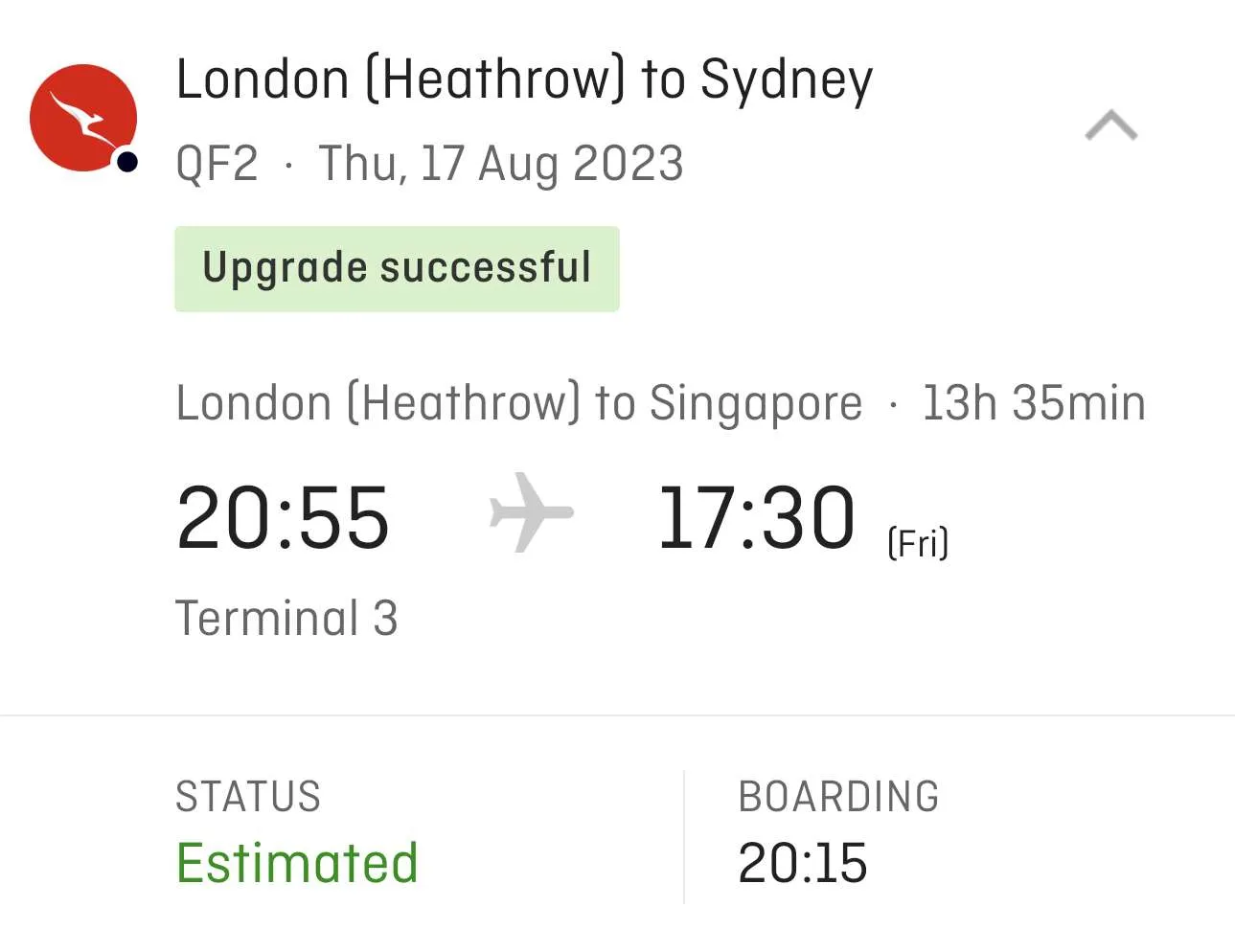A screenshot of flight information is displayed on a pristine white background with black text, showcasing a traveler's journey from London Heathrow to Sydney on Thursday, August 17th, 2023. Prominently, a green box with black text indicates "Upgrade Successful." The itinerary details a segment from London to Singapore, highlighting a flight duration of 13 hours and 35 minutes. Departure is listed from Terminal 3 at 20:55, with an arrival in Singapore at 17:30 on Friday. A small airplane icon sits between the departure and arrival times. Below this, gray text reads "Status," followed by green text stating "Estimated." Adjacent to this is gray text denoting "Boarding" with the boarding time of 20:15 written in black. The layout is clean and highly readable, featuring large, easily decipherable text. In the top left corner, a red and white logo with a small black dot adds a touch of color to the otherwise monochromatic display.